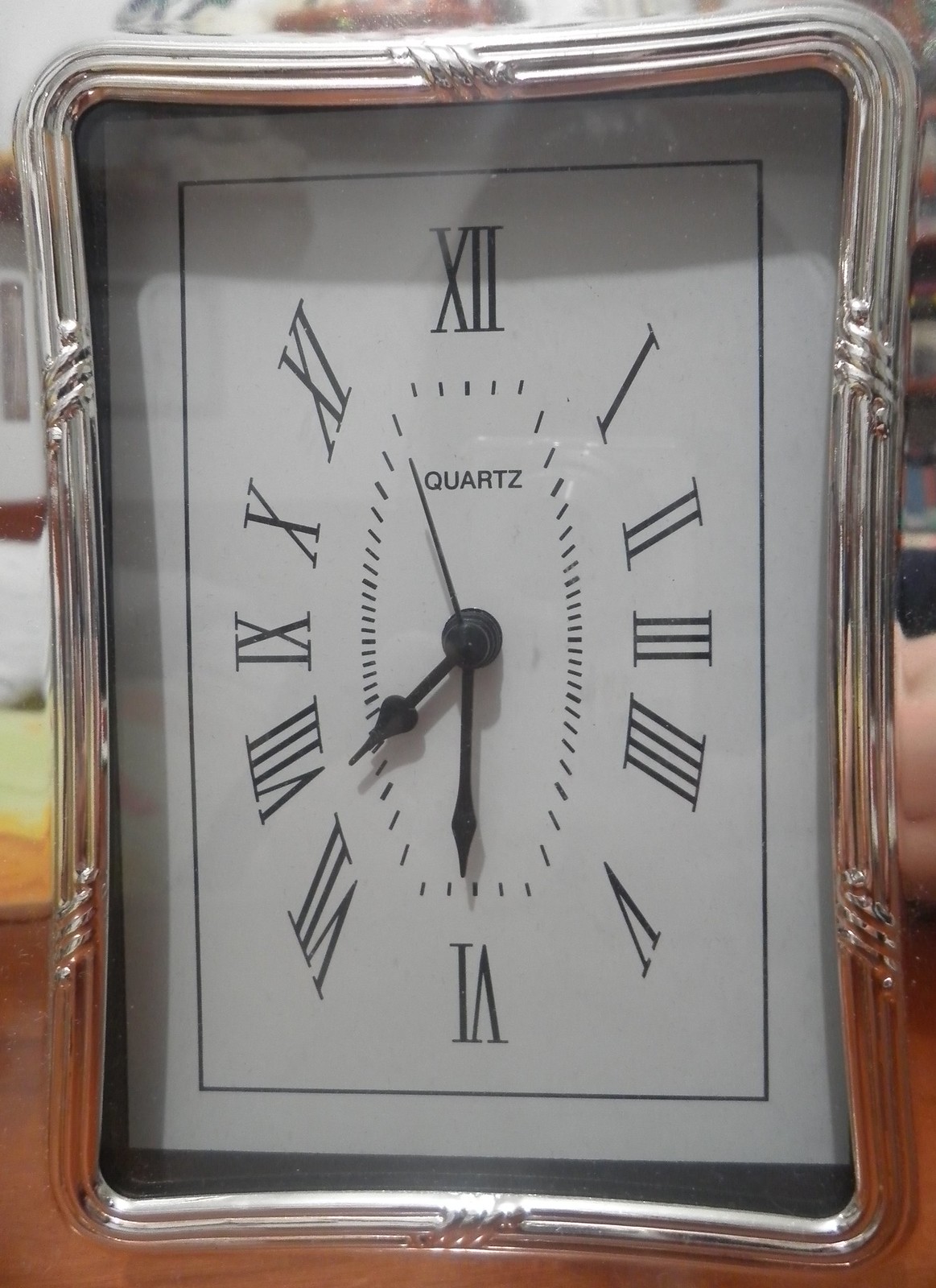The image features a distinctive desk clock with a silver frame and a white face covered in glass, reflecting light. The clock is designed with Roman numerals in black and black hands, indicating a time of approximately 7:30, with the second hand positioned just past 11. Notably, the clock has an elongated shape that is taller than it is wide, with rounded corners and a distinctive dip along the sides. The word "Quartz" is prominently displayed above the hands. The clock is situated on a brown wooden surface, adding to the overall aesthetic with a mix of reflections and surrounding colors in the background. The design, though unusual, gives the clock a charming and elegant appearance.